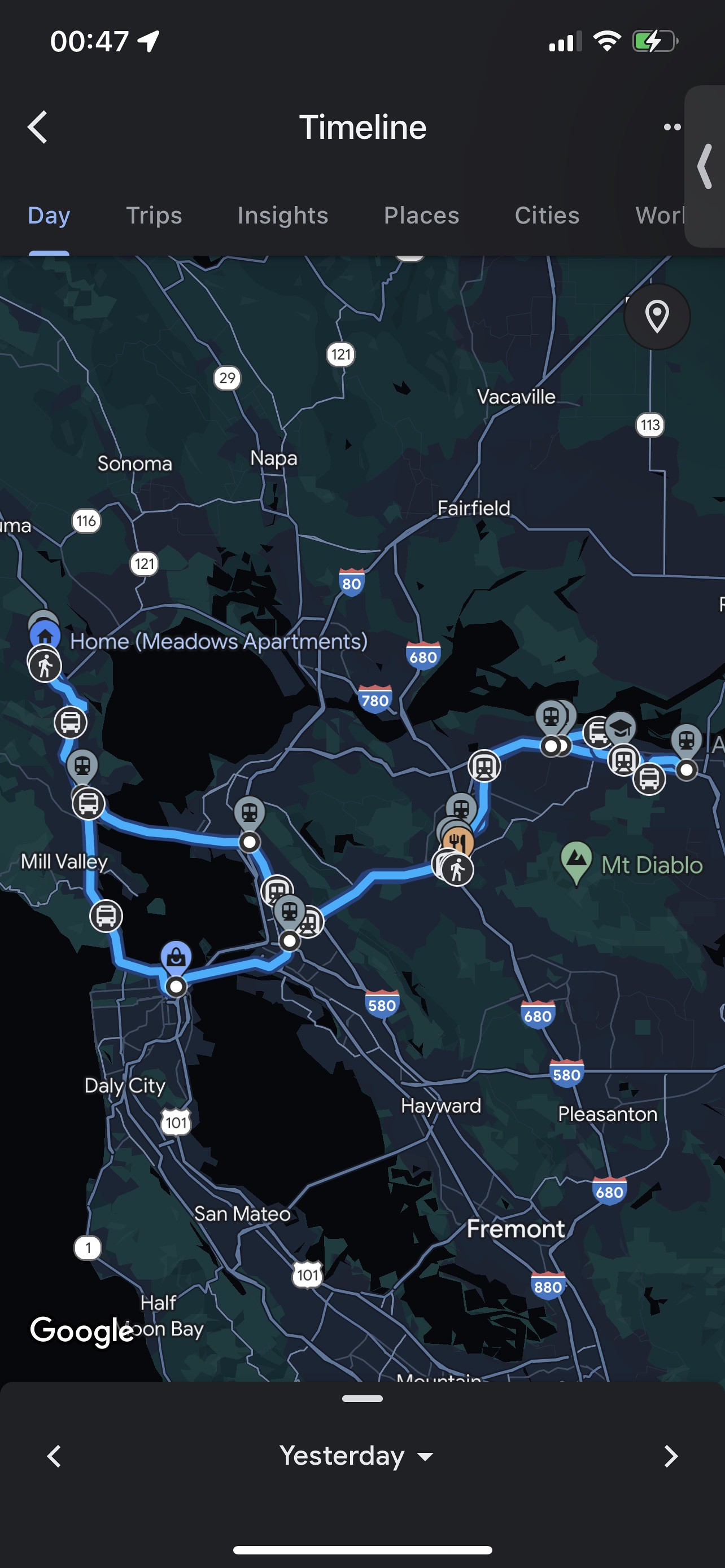This horizontally-oriented image is a detailed screenshot of a smartphone displaying a travel planning map. The map occupies the majority of the screen, bordered by black strips at the top and bottom. The top strip features the current time on the left and battery and Wi-Fi signal indicators on the right. Flanking the top banner are scroll arrows on both sides. The banner reads "Timeline" with subsections labeled "Day," "Trips," "Insights," "Places," and "Cities," with a highlight under "Day," indicating it is currently selected.

On the bottom black strip, the word "Yesterday" appears in white text, also accompanied by scroll arrows at both ends. The map itself illustrates a planned route marked by a light blue line, traversing various interstate highways and stopping at different key points. Icons representing different types of transportation and food locations punctuate the route. A notable location, "Mount Diablo," is marked in green, signifying its natural significance or attraction status. This map showcases someone's detailed travel itinerary, meticulously inputted into their smartphone.